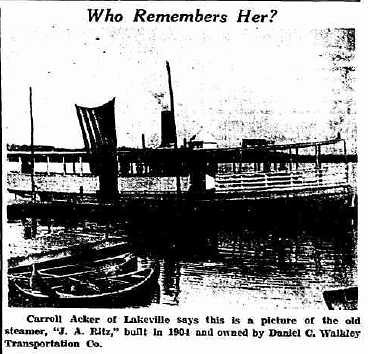This black and white image, reminiscent of an old newspaper snippet, prominently features the historic steamer J.A. Ritz, built in 1904 and owned by the Daniel C. Walkley Transportation Company. Centered in the photo, the boat rests on the water, flanked by two smaller boats, one of which is tied to a dock in the left foreground. The grainy texture and monochromatic palette emphasize the photograph's vintage nature. Text overlays the top and bottom of the image, with the upper caption reading, "Who Remembers Her?" and the lower text attributing the picture's identification to Carol Acker of Lakeville. The outdoors setting adds to the nostalgic and historic ambiance of this well-worn image.